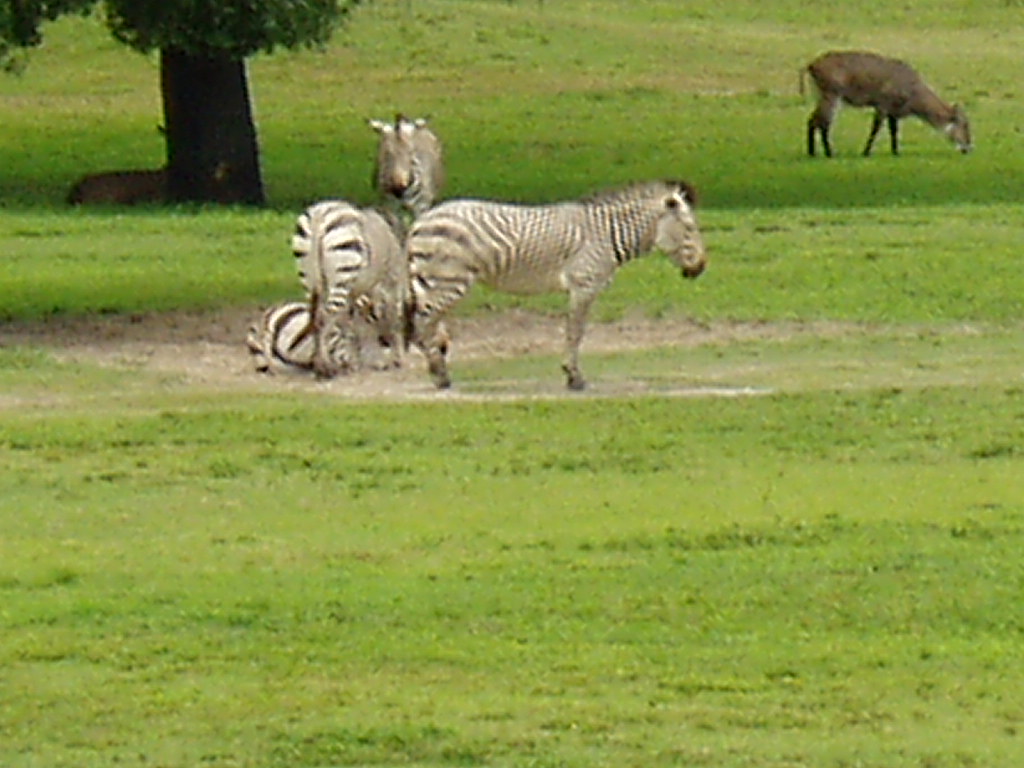This slightly grainy, horizontally-oriented color photograph captures a lively outdoor scene of a grassy field, possibly part of a zoo or a natural prairie habitat. At the center of the image, four zebras occupy a patch of dirt amid the lush green grass. One zebra stands sideways, offering a clear view of its black and white stripes, while another zebra stands with its back to the camera. A third zebra faces the camera directly, and the fourth zebra is laying down, its tail end visible.

In the background, towards the upper right corner, stands an unidentified brown mammal, possibly a deer or gazelle, grazing on the grass. On the left side of the photograph, a large tree trunk with dense green leaves is visible, casting a shadow on the ground. Another animal, partly obscured and reclining against the tree, hints at either large ears or horns.

The picture is taken during daylight, with ample sunlight illuminating the scene, and shows a slightly blurred, low-resolution quality, characteristic of a telephoto lens image. The natural setting depicted adds to an overall tranquil and observational mood.